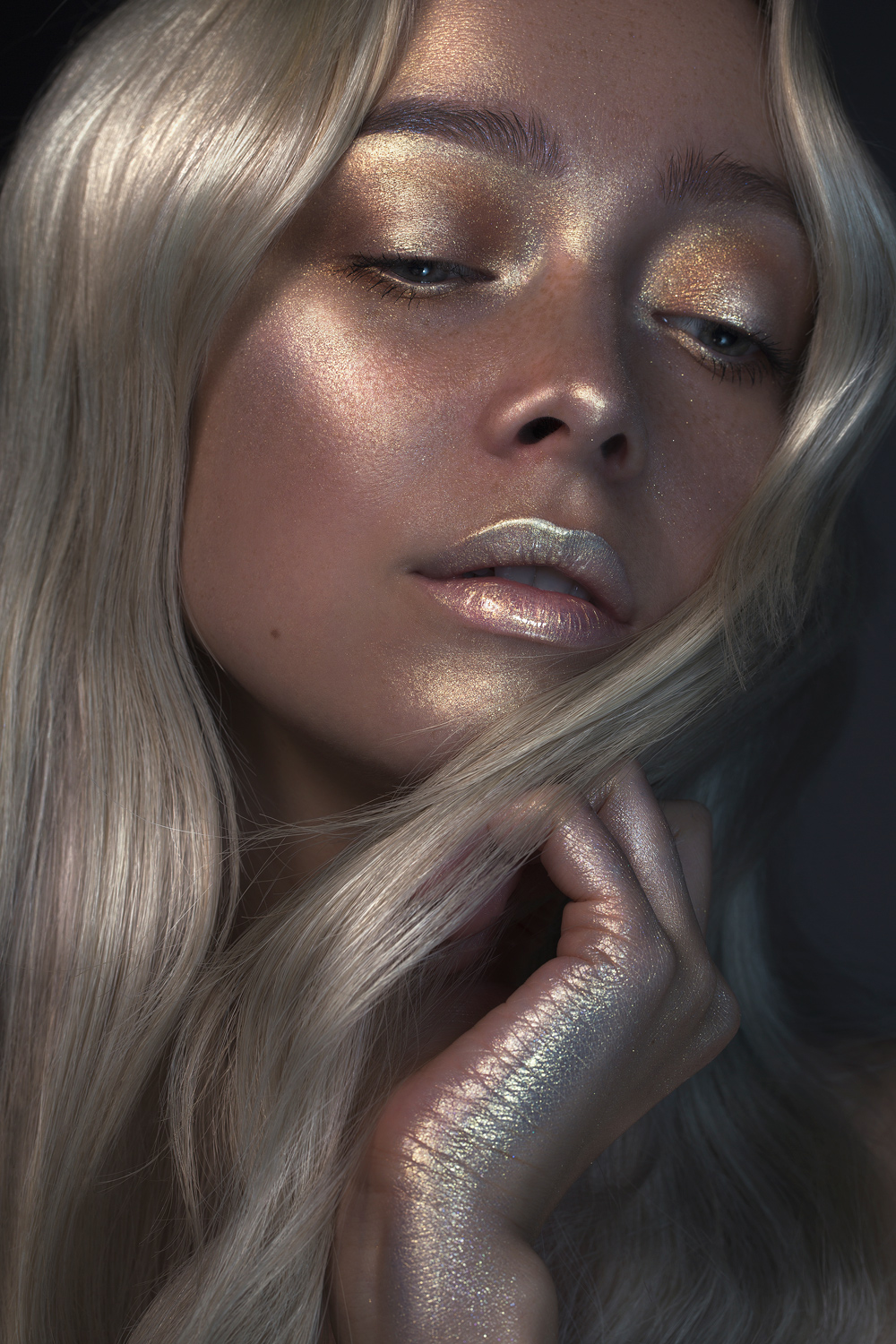This is an image of a young woman with long, flowing blonde hair, captured against a black background. Her face, hand, and lips are covered in a glittery, metallic material that emits a bronzy reflection, lending an ethereal, rainbow-like sheen to her complexion. She has darker skin, accentuated by the highlighter that shines intensely on key points such as her eyelids, cheeks, the tip of her nose, and the middle of her brow. Her eyes appear to be brown, with her eyebrows a shade darker than her hair. She is gazing downwards and to the right, her expression one of contemplation or solemnity. Her right hand is gently resting under her chin, also adorned with the glittery substance. Her mouth is partially open, revealing a glimpse of her teeth, and her lips are notably shinier and more glittery at the top. The overall effect is enhanced by what appears to be digital or filter enhancements, making the shimmering detail even more pronounced.